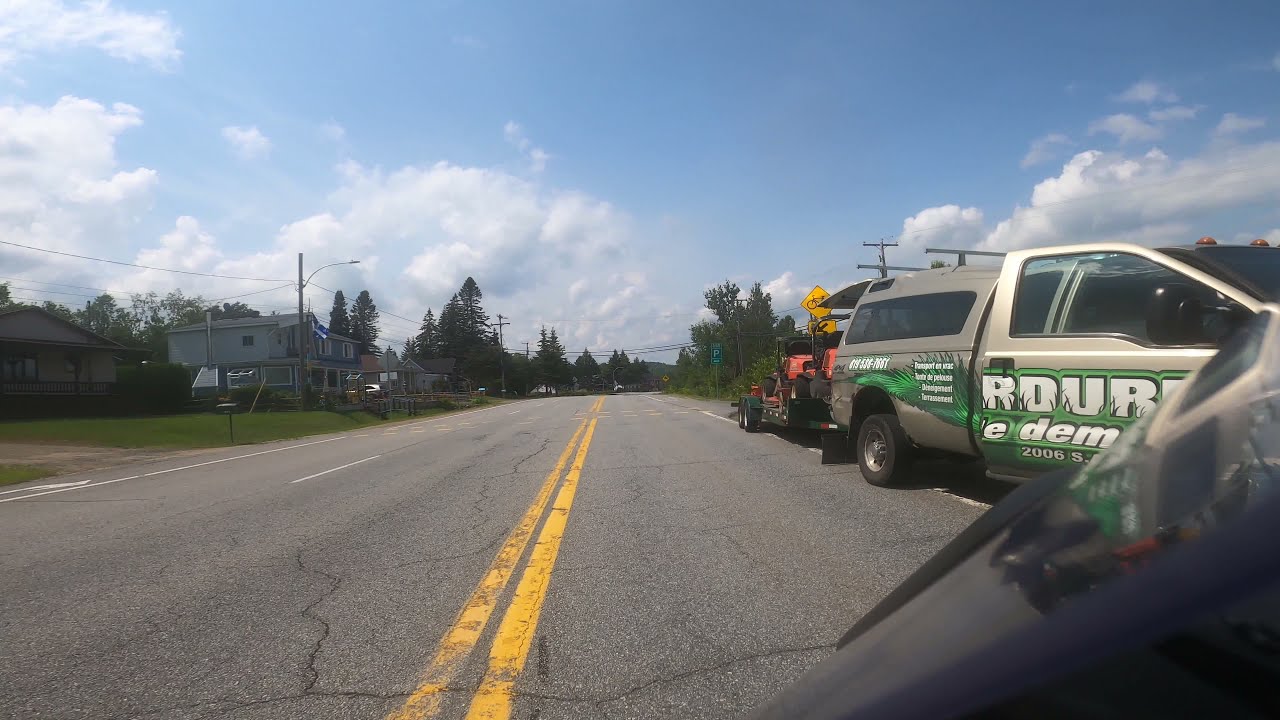This image captures a first-person view of a long, gray road marked with dual yellow lines separating traffic. The scene unfolds during daytime under a vast blue sky adorned with multiple white clouds. On the left side, power poles and streetlights line the road, with grass patches leading up to several buildings, including a noticeable gray two-story house. In the distance, pine trees frame the view on both sides.

Dominating the right side of the road is a silver truck with green and white writing on its side, potentially in another language. This truck appears to be a business vehicle, likely for landscaping, given the presence of red riding mowers and a trailer attached behind it, carrying orange tractors. The truck’s passenger door is open. A yellow street sign and various cracks on the road surface are also visible, adding to the detail of this outdoor snapshot. A car is hinted at in the foreground, partially visible and blurry.